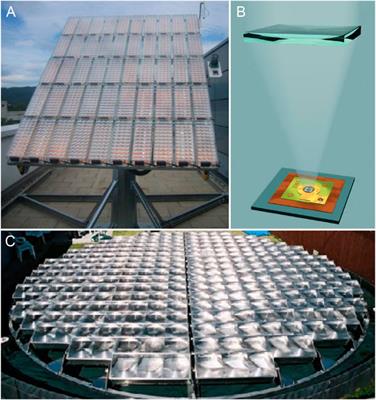The image is a composite of three labeled photographs, identified as A, B, and C. Photograph A, located on the top left, depicts a rectangular rooftop solar panel set against a sky background. This panel features an array of smaller diodes and is mounted on a stand, appearing to harness solar energy, possibly radiating heat. Photograph B, situated on the top right, seems to be an illustration rather than a photograph. It showcases a flat, square tile with concentric regions of teal, rusty red, and a yellow-green center. A beam of light extends from the center of this tile, forming a cone shape aimed at the teal rectangle above, suggesting a demonstration of stored energy radiation. Photograph C, occupying the bottom section, portrays a large, reflective circular grid composed of multiple rectangular sections. This round structure, with its shiny, silver appearance, might function as a heat control mechanism or be purely decorative, laying flat on a surface and resembling a solar array.